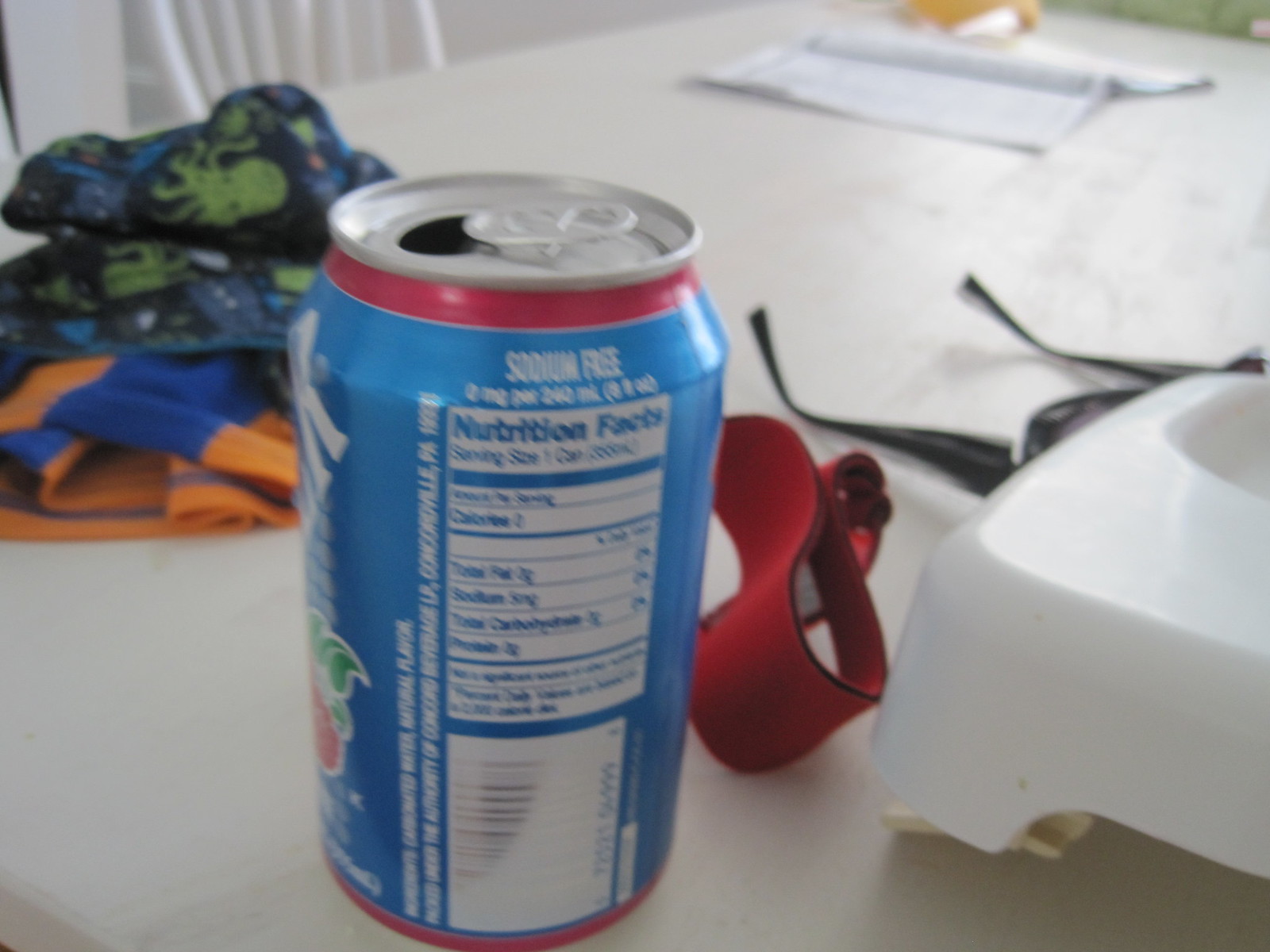This slightly blurry photograph captures a cluttered white desk or table. In the foreground, there is an open soda can with a blue label accented by red rings at the top and bottom. The can is positioned in such a way that the Nutrition Facts label is prominently visible, obscuring any branding. Positioned behind the can, a red strap lies on the table, hinting at a possible accessory. To the left of the strap, a piece of fabric in a striking orange and blue color scheme adds a splash of vibrancy. Above the fabric, there is an item with an intricate design, though its details are somewhat unclear. On the right side of the image, the arms of a pair of glasses are visible, partially obscured and lacking visibility of the lenses. In the background, there is an open magazine or book, adding to the sense of a busy, multi-purpose workspace.